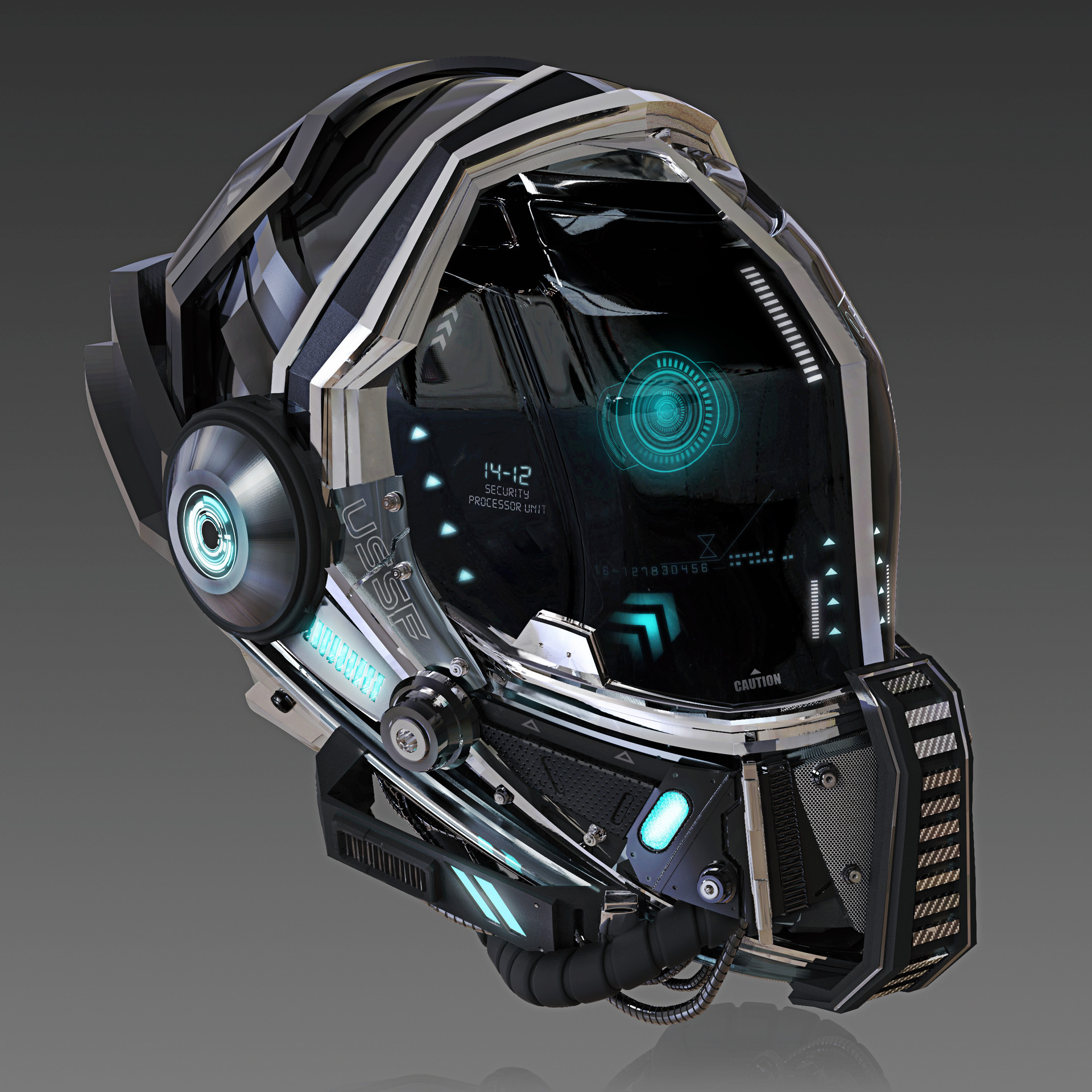This is a detailed render of a highly complex, futuristic helmet, reminiscent of those seen in sci-fi video games such as Mass Effect. Predominantly black and shiny, the helmet features intricate details and advanced technological elements, suggesting it could be designed for space or hazardous environments. Emerging from its base are black tubes that extend and connect to the back of the helmet, giving it a robust and utilitarian appearance. A prominent silver disc and a logo reading "USSF" are visible on one side, hinting at a possible affiliation with a futuristic space force. The visor, a sleek black faceplate, displays a sophisticated heads-up display (HUD) with teal-colored elements, including a glowing ring with radial bars and a central circle, as well as directional arrows and text that reads "1412 security processor unit." This HUD is likely designed to convey critical information to the wearer, such as oxygen levels and environmental conditions, underscoring the helmet's advanced, high-tech functionality.